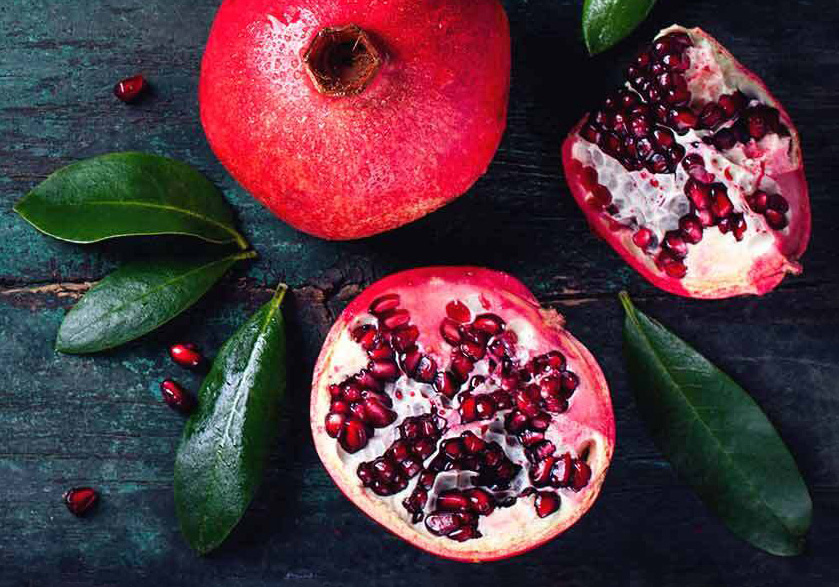This indoor color photograph captures a vibrant still life of pomegranates on a dark, age-worn wooden table, painted in a blackish-green hue. At the center of the composition lies a whole, deep dark red to purple pomegranate, its glossy skin contrasting with the rugged surface beneath. Surrounding it, a sliced pomegranate reveals a cluster of gleaming red seeds within its rich, pulpy interior. One slice is centrally placed, while another rests in the top right corner. Scattered across the scene are five long, thick green leaves, artfully arranged around the fruit - three on the left side of the central slice, and two more at the top right and bottom right corners. Enhancing the rustic charm, several loose seeds glisten on the table, with three positioned at the bottom left and one near the top left. The meticulous arrangement underscores the natural beauty and vibrant color palette of the fruit and foliage, set against the textured backdrop of the wooden surface.